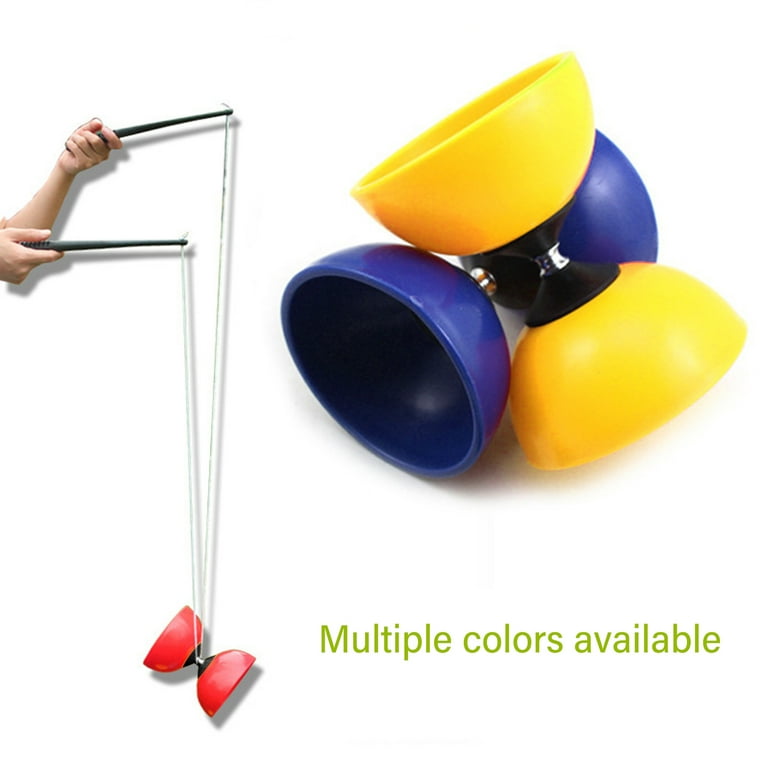The image is a meticulously staged and edited collage made up of several full-color photographs, laid out in a borderless, square format against a white background. Centered to the right in bright green text, it states, "Multiple colors available." Dominating the right side, the image features a toy composed of two yellow and two blue shiny, semicircular plastic pieces, connected in the middle by a black element, resembling stacked bowls or lids. Two Caucasian hands are holding brown sticks, each connected by a string forming a loop that supports the toy. The configuration suggests the toy operates by manipulating the sticks to control the device's movement, likely allowing it to be balanced or tossed into the air and caught again.